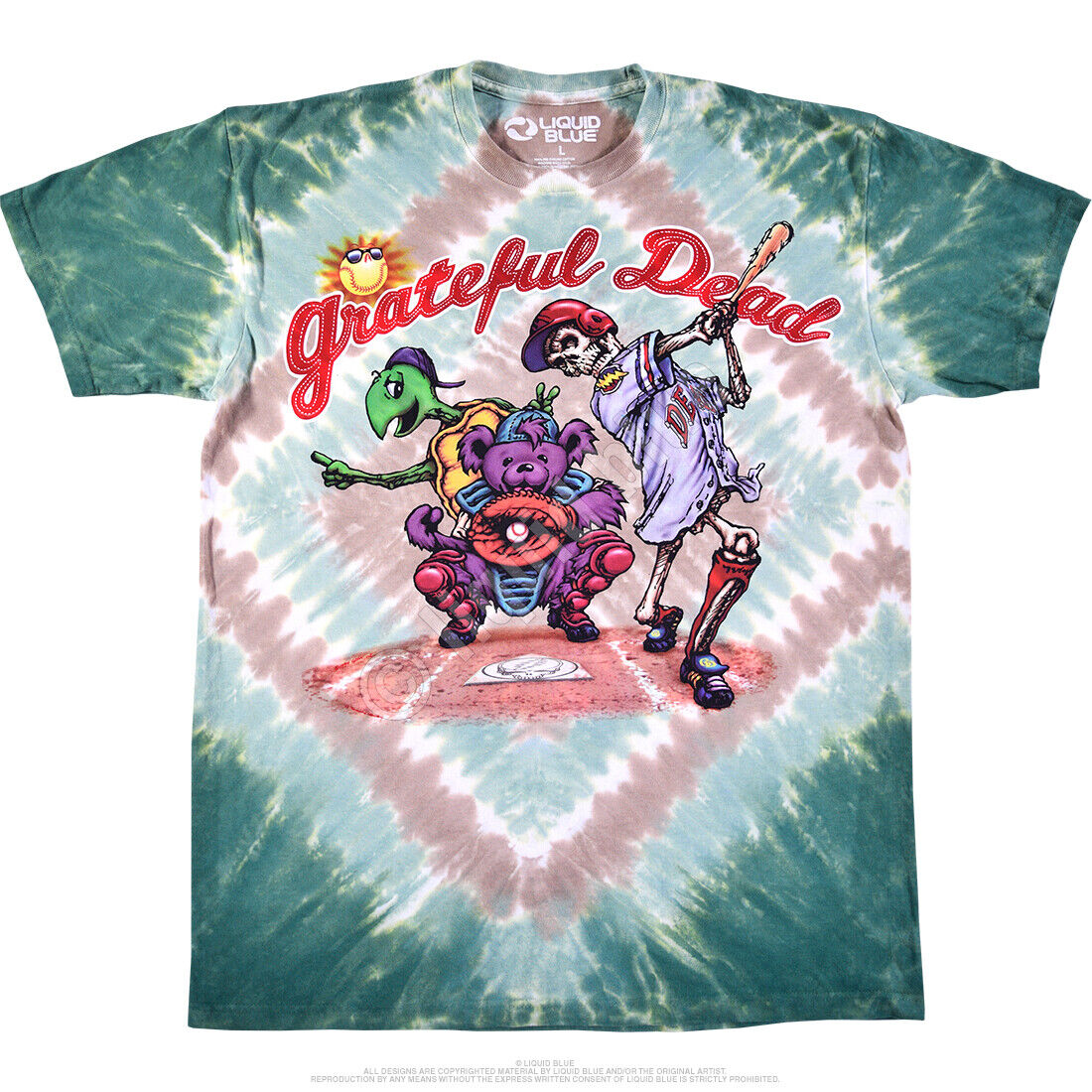This image is a color photograph in portrait orientation featuring a detailed crewneck, short-sleeved tie-dye t-shirt. The t-shirt, size large and produced by Liquid Blue, showcases an elaborate tie-dye pattern with a dark teal-blue background, a rose-colored diamond inset, light aqua accents, and green and white highlights on the sleeves and base. At the center of the t-shirt, the headline "Grateful Dead" is written in red script, arcing across the top. Above the "RNA" in "Grateful," a stylized sun, adorned with sunglasses and resembling a smiling baseball, draws attention. The central graphic depicts an animated skeleton baseball player at home plate. The skeleton, clad in a gray baseball shirt, red helmet, and red knee socks with cleats, smiles down at the ground, having missed a swing with its bat raised in the air. Beneath its feet is a red dirt base with a white home plate. Behind the skeleton, a purple bear functioning as the catcher wears a blue safety vest, complete with knee pads and a catcher's mitt in orange, holding the baseball triumphantly. To the left of the bear, a turtle dressed as an umpire, shown in profile with a backwards black cap, points decidedly to the left, making a call. The shirt embodies a vivid realism with animated figures, merging elements of both fashion photography and representational art.